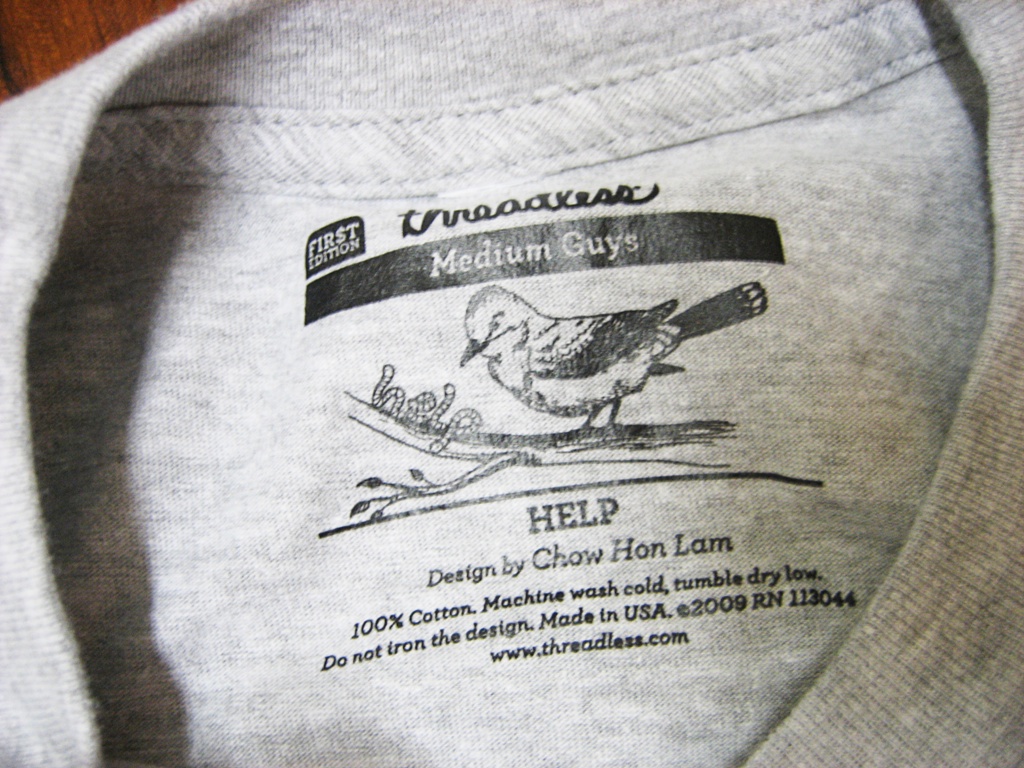This image showcases a light gray crewneck sweatshirt. The photograph specifically focuses on the printed tag located on the inside of the garment, rather than the entire sweater. The text on the tag is displayed in black and white and features several informative details. 

At the top of the tag, it reads "First Edition," followed by "Threadless," indicating the brand. The size is labeled as "Medium," specifically targeting guys. Below this, there is a detailed sketch of a bird perched on a branch with worms in front of it, seemingly getting ready to eat them.

Underneath the bird sketch, the text states "Help design by Chow Han Lam," giving credit to the designer. Additional care instructions are provided: "100% cotton, machine wash cold, tumble dry low, do not iron the design." The tag also indicates that the sweatshirt was made in the USA in 2009, with the RN number 113044. Lastly, the website "www.threadless.com" is listed for further reference.